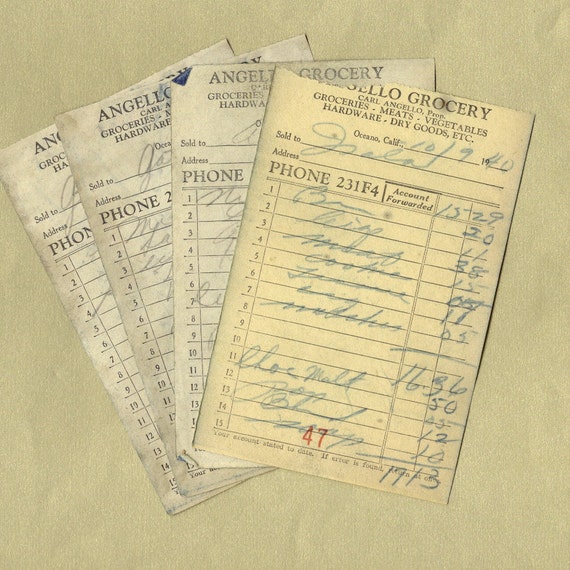This photograph captures four aged grocery receipts from Angelo's Grocery, meticulously laid out on a plain gray ivory background. Each receipt, yellowed with time and some torn, is written in cursive ink. The recurring header on all receipts reads: "Angelo Grocery, Carl Angelo, Proprietor: Groceries, Meats, Vegetables, Hardware, Dry Goods, etc." Dated October 9, 1940, the receipts list items like eggs, cookies, chocolate malt, bread, and chocolate milk, with individual prices noted on the far right and a total at the bottom. The receipts are arranged in a fanned-out manner, revealing that three are on white paper while one on the far right is distinctly yellow. The predominant hues in the image include shades of gray, tan, and faded yellow, reflecting their age and historical charm.